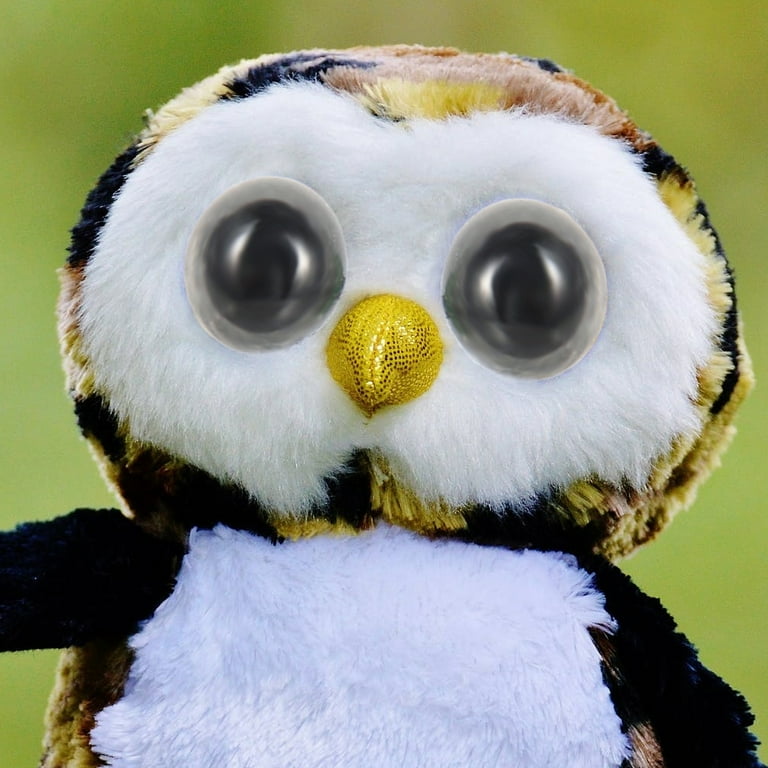This photograph captures a charming T.Y. plush toy, designed to delight children with its vibrant and whimsical appearance. The toy depicts an owl with endearing, oversized black eyes that evoke a sense of innocence and curiosity. Its bright yellow beak, adorned with shimmering gold foil accents, glitters and draws immediate attention. The plush owl's "feathers" are crafted from an assortment of faux fur in a medley of colors, including yellow, brown, tan, and black, giving it a rich and textured look. Surrounding the eyes and covering the chest area is a contrasting white faux fur, adding a touch of softness and highlighting the owl’s facial features. Set against a backdrop of varied light green shades, the image suggests an outdoor setting, likely in front of a bush or tree, enhancing the natural and playful aesthetic of the plush toy.